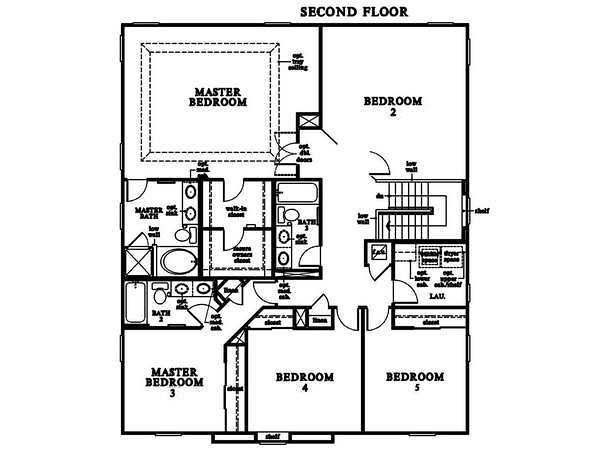The image showcases a detailed blueprint of the second floor of a house, depicted in black outlines and lettering. In the upper right-hand corner, the label "Second Floor" is prominently displayed. 

On the top left-hand side, the "Master Bedroom" is clearly labeled, adjacent to "Bedroom 2" on the right. Both rooms are shown with their respective closets and doorways. Beneath these rooms, starting again from the left, the "Master Bath" is labeled and includes an illustration of the doorway. 

Continuing to the right, two walk-in closets are depicted, followed by another bathroom. Below these features are additional bathroom spaces. At the bottom of the blueprint, the rooms labeled "Master Bedroom 3," "Bedroom 4," and "Bedroom 5" are shown, completing the detailed floor plan.